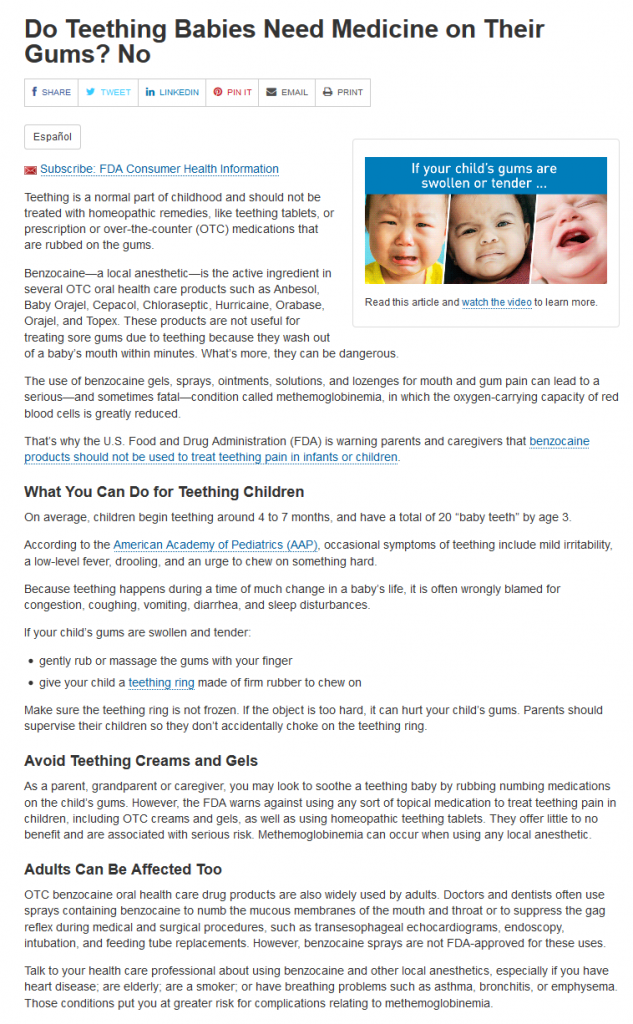This image is a screenshot of a website with a white background. At the top, a headline in large, bold, black lettering reads, “Do teething babies need medicine on their gums? No.” Directly beneath this, there are buttons for sharing the article on Facebook, Twitter, LinkedIn, Pinterest, via email, and for printing. There is also a button below these options for translating the article into Spanish.

On the right side of the page, there is a small inset color photo of three babies crying. Text overlaying this image instructs, “If your child's gums are swollen or tender, read this article and watch the video to learn more.”

The article itself comprises multiple paragraphs, with all the text in black and certain portions highlighted as blue hyperlinks. It begins by explaining that teething is a natural part of childhood and advises against using homeopathic remedies like teething tablets or any medications, prescription or over-the-counter, that are intended to be rubbed on the gums. The article specifies that benzocaine—a local anesthetic found in several over-the-counter oral care products such as Anbesol, Baby Orajel, Cepacol, Chloraseptic, Hurricane, Orabase, Orajel, and Topex—is not effective for treating teething pain because it washes out of a baby’s mouth quickly. Furthermore, it underscores the potential dangers of these products, explaining that benzocaine gels, sprays, ointments, solutions, and lozenges can lead to a serious, sometimes fatal condition known as methemoglobinemia, where the oxygen-carrying capacity of red blood cells is greatly reduced.

The article continues by listing safer alternatives and remedies for teething children, advising against the use of teething creams and gels, and also addresses how adults can be affected by these products.